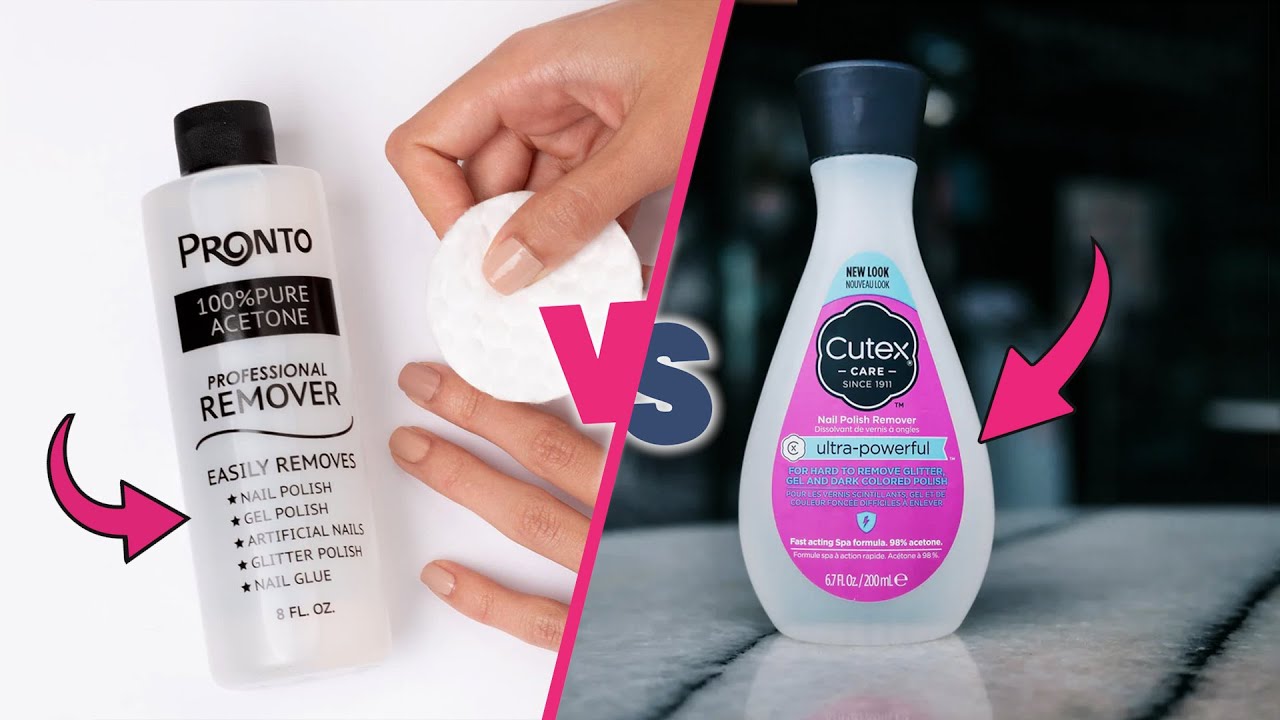In this image, we see a comparison between two types of nail polish remover, presented side by side. The left half features a cylindrical, clear plastic bottle with a black cap, branded as Pronto. This bottle, labeled 100% pure acetone, professional remover, claims to effectively remove nail polish, gel polish, artificial nails, glitter polish, and nail glue. The text also mentions an 8 fluid ounce capacity. A pink arrow points towards this bottle, and there is an image of a person using a round cotton pad to apply the remover. Separating the two images is a vertical pink dashed line with a large "V" on it, signifying "versus."

On the right side, we have a teardrop-shaped bottle, also plastic with a black cap, labeled as a Q-tips Care product. This bottle advertises a "new look" and touts itself as ultra-powerful, designed for removing hard-to-remove glitter, gel, and dark-colored polish. The text provides details in both English and French, emphasizing its fast-acting spa formula with 98% acetone content and a 6.7 fluid ounces capacity. A pink arrow also points towards this bottle, mirroring the style on the left side. The entire composition highlights the comparative nature of the two products, focusing on their packaging and efficacy claims.